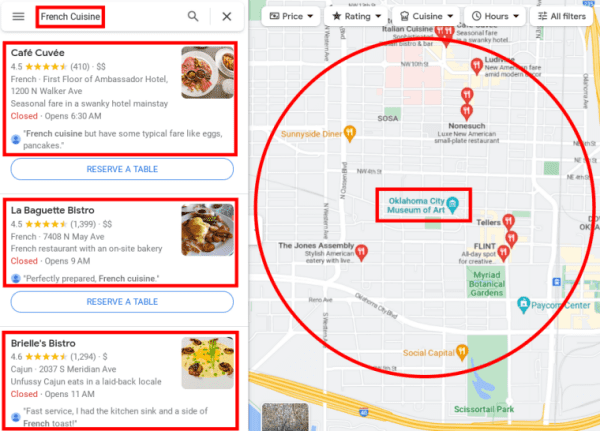**Category: Websites**

The image showcases a detailed map on the right-hand side, with a notable red circle delineating a specific area. Within this red circle, several restaurants are highlighted with map points, marked in either red or yellow colors, indicating various categories or statuses. All restaurants shown fall within a certain radius on the map, although it does not specify the exact location.

On the left side of the image, there is a search engine interface with a highlighted red box around it, prominently displaying the search term "French cuisine." Below the search field are a couple of search results:

1. **Café Cuvée**: Rated 4.5 stars, located on the first floor of the Ambassador Hotel at 1200 Walker Ave. The restaurant is currently closed and will open at 6:30 a.m. It offers French cuisine with some typical breakfast items like eggs and pancakes. There is an option to reserve a table available.

2. **La Baguette Bistro**: Also rated 4.5 stars, situated at 7408 North May Avenue. This French restaurant features an on-site bakery. It is currently closed and will reopen at 9 a.m.